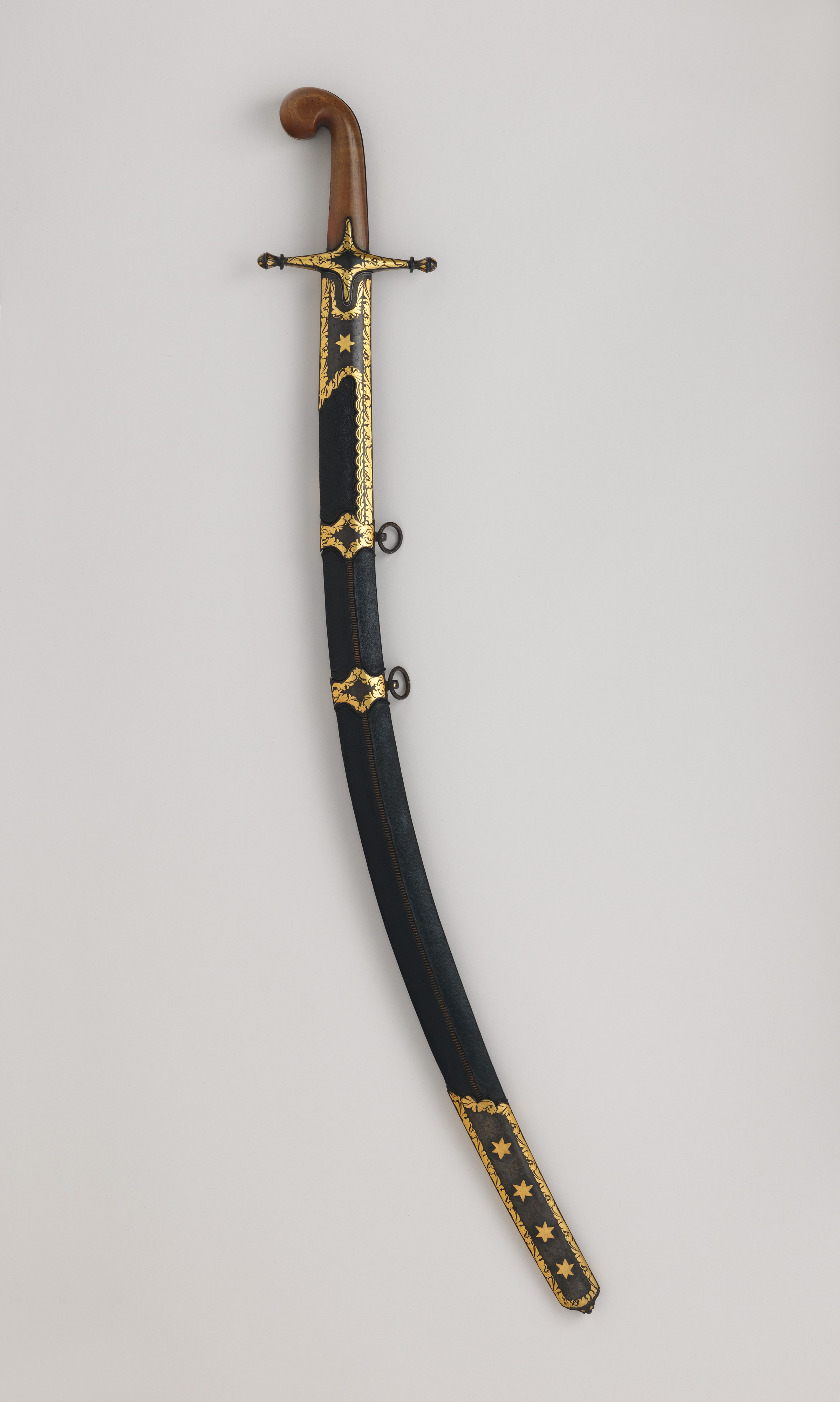This image is a professionally taken product photograph of a sheathed katana displayed against a plain light gray or white background. The katana's sheath features intricate gold and black designs, giving it a distinct fantasy aesthetic. At the bottom of the sheath is a prominent gold star surrounded by detailed etchings, with additional gold accents that stretch upwards towards the top. These gold accents include six-point and four-point stars, adding to the weapon's elaborate decoration. The sheath has a luxurious black finish that resembles black laminate wood, while the gold appears shiny and metallic. The weapon's handle, situated at the top, is made of wood and complements the overall design. The katana's blade, though not visible, is suggested to be curved. The photograph is minimalist yet detailed, ideal for showcasing the katana, possibly for retail purposes.